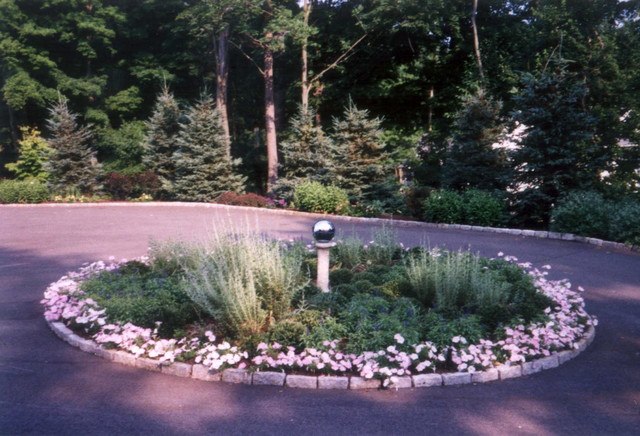This full-color, outdoor photograph, taken during the day with natural light, features a square image dominated by trees in the upper half, with smaller pines in the foreground and larger hardwoods further back. The top edge reveals a glimpse of blue sky. In the lower half, there's a decorative planter set within a circular drive, likely part of a residential setting. The planter is bordered by white bricks and contains small plants and flowers, framing a central white pillar topped with a reflective silver ball. Surrounding the planter, you can see patches of gray asphalt, indicating the circular drive that encircles the planter. The drive outlines the image from the middle left to the middle right, curving slightly. Dense woodland, particularly pine trees, forms a scenic backdrop beyond the drive, creating a serene and picturesque scene.